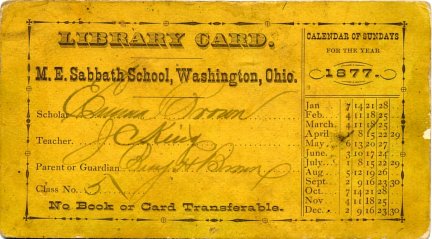This vintage library card, printed on a dark yellow, rectangular piece of paper, features a thin faded black border surrounding its edges. The card, which is longer horizontally than vertically, shows signs of wear, including a noticeable stain on the right side. At the top, in block letters, it proudly states "Library Card." Below this, it reads "M.E. Sabbath School, Washington, Ohio." The card is organized into sections with text and lines for signatures, all written in pencil. The sections labeled "Scholar," "Teacher," and "Parent or Guardian" each have an illegible cursive signature beside them. Additionally, it is marked with "Class Number: five" and a cautionary notice that "No book or card transferable." Finally, on the right side, a column is dedicated to a "Calendar of Sundays for the year 1877," listing the months vertically along with corresponding dates.